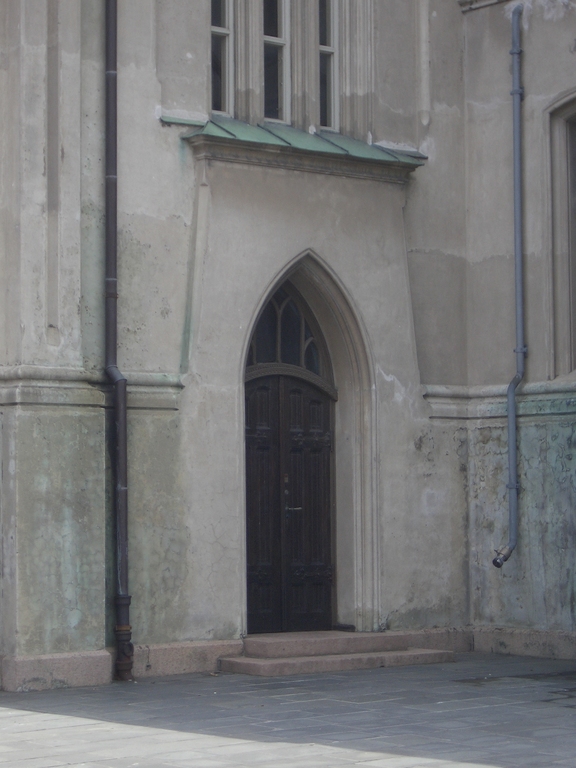This color photograph captures the entrance of a church-like building with a distinctive design and intricate details. The focal point is a tall, narrow, slightly pointy doorway, shaped like an elongated arch, reminiscent of gothic architectural style. The door itself is crafted from rich, dark cherry wood, adorned with a small handle. Surrounding the doorway are beige cement or stone walls that lend an aged, somewhat faded appearance to the structure.

There are two stone steps leading up to this entrance, suggesting it might be a side entrance rather than the main one. Above the door, three slender windows are vertically aligned, emphasizing the building's towering height. Directly below these windows is a small green roof or balcony, although it appears too fragile for use.

Flanking the door are pipes running vertically along the walls, likely serving as rain gutters. The pipe on the left is dark brown, while the one on the right is a silver metal color. One of these also functions as a water tap. The overall scene is set in a stone-paved yard, casting a grey shadow on the ground, with a strip of sunlit ground visible on the left side.